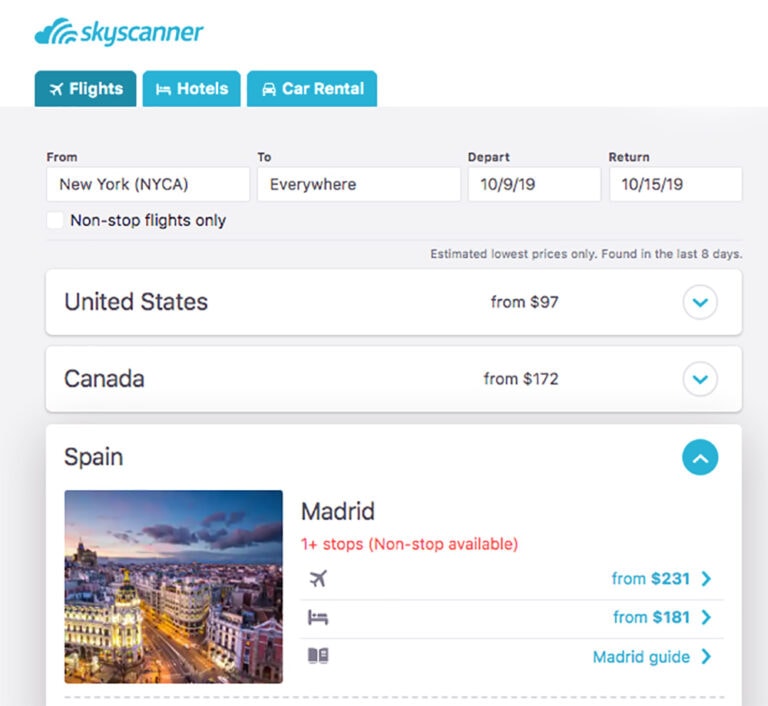This screenshot, taken from the Sky Scanner app or website, prominently displays the blue Sky Scanner logo at the top. Below the logo are three blue tabs labeled "Flights," "Hotels," and "Car Rental." The search fields show a "From" text box with "New York, NYCA" entered and a "To" text box with "Everywhere" as the input. The search parameters include a departure date of 10/9/19 and a return date of 10/15/19. 

A box for selecting "non-stop flights only" is present but remains unchecked. The section below lists "Estimated Lowest Prices" found in the past eight days: flights from the United States start at $97, from Canada at $172, and to Madrid, Spain with one or more stops at $200. Non-stop flights to Madrid are also available starting at $231. The information also indicates that hotel prices in Madrid begin at $181. Additionally, there's an option to access a "Madrid Guide."

To the left of the screen, there's an aerial view of Madrid with dramatic stormy skies in the background. The city is illuminated, creating a striking contrast against the cloudy backdrop.